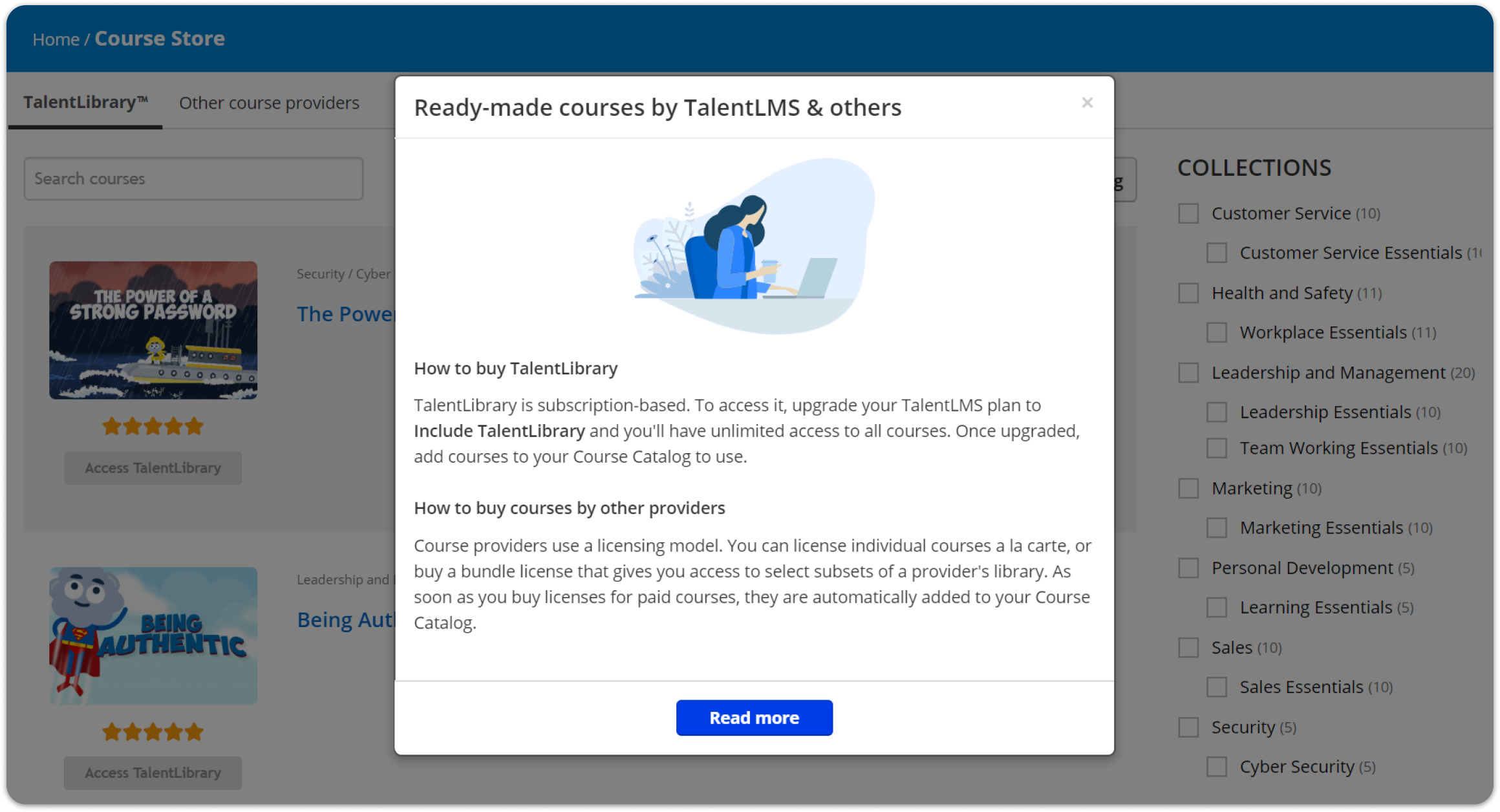**Title: How to Access Talent Library on Talent LMS**

The screenshot showcases a detailed guide within an app—possibly a web page—viewed on a tablet in landscape mode. The background is grayed out, accentuating a prominent pop-up window with rounded corners. The header titled "Ready-made courses by Talent LMS and others" informs users about the featured content. In the upper right corner, there's a conspicuous 'X' for closing the pop-up.

Beneath the header, there is a detailed vector graphic depicting a serene scene with a young woman seated comfortably in a chair. She appears to be typing on her laptop with one hand, while the other hand is holding a glass. The backdrop consists of various shrubs and greenery, creating a calming and studious ambiance.

The text below offers guidance on purchasing the Talent Library. It explains that the library operates on a subscription model, and users must upgrade their Talent LMS plan to gain unlimited access to all courses within the Talent Library. To integrate new courses into your catalog, it is necessary to either select individual courses à la carte or purchase a bundled license that includes a subset of the provider's offerings. Once licenses for paid courses are acquired, they are automatically added to your course catalog.

At the bottom of the pop-up, a blue button labeled "Read More" invites users to delve further into the subject.